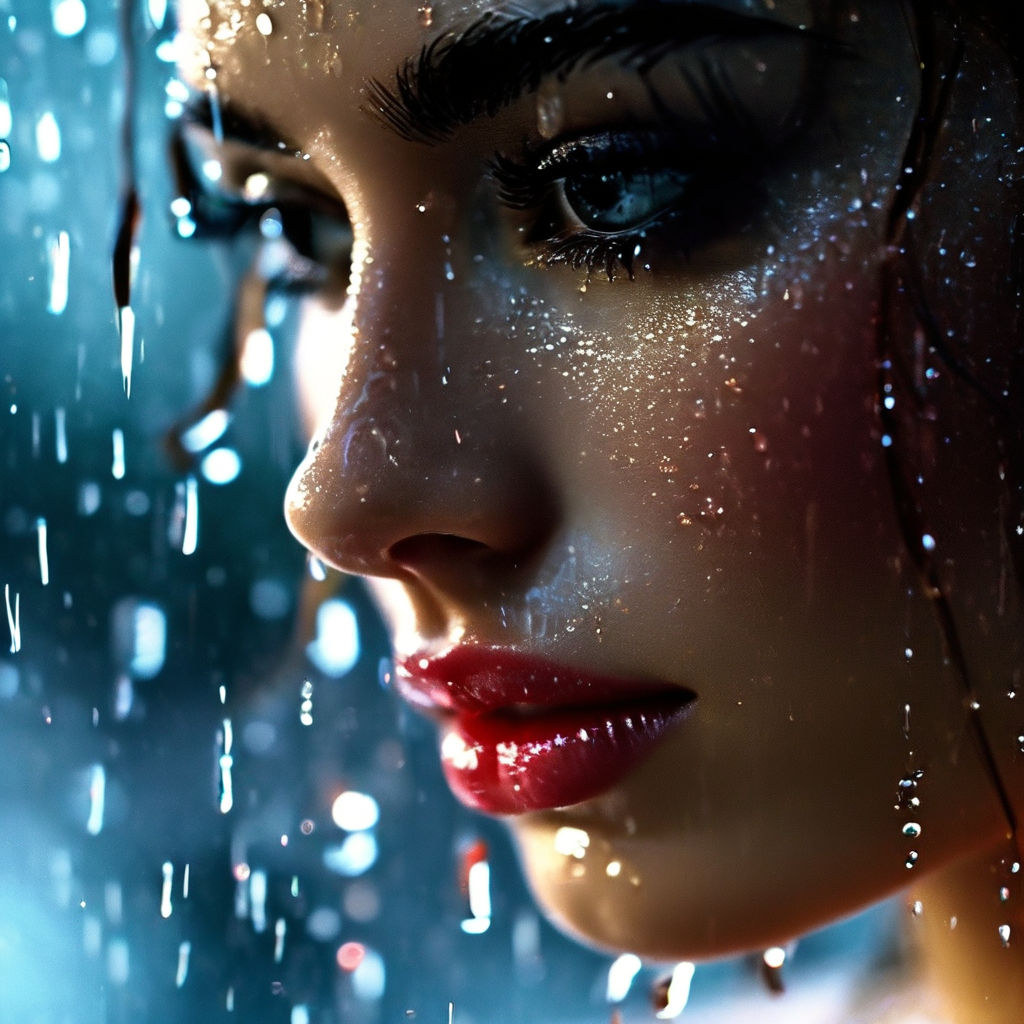The image is a high-resolution, professionally rendered photo of a woman, her face adorned with full makeup and mid-rainfall. She has striking, bushy eyebrows and long lashes coated in waterproof mascara, eyeshadow adding a shimmer to her eyelids, and bold, wet-looking red lipstick. Her hair, soaked by the rain, clings to her face, while each water droplet glistens under high-contrast lighting that accentuates one half of her face, rendering the other side in shadow. The woman’s expression is blank and emotionless, perhaps hinting at sadness or anxiety, her eyes reflecting the grayish-blue ground below. The backdrop is a blurred mix of blue hues, contrasting sharply with her orange-tinted skin. Despite the rain, every detail from the makeup to her perfectly styled yet wet appearance gives the impression of a meticulously staged magazine ad. Her ethnicity appears to be ambiguous, potentially Caucasian, Hispanic, or Middle Eastern, adding an element of mystery to her striking presence.